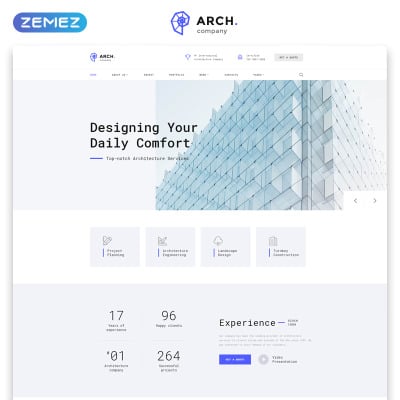This detailed caption encapsulates the various elements of the image in a descriptive manner. Here it is:

---

The image appears to be a screenshot from a website, likely an advertisement or promotional material for a company. At the top left corner, it features the word "ZMEZ" written in all capital letters using a digital clock-like font, composed of single bars. The text "ZMEZ" is in white, positioned on a blue oblong background. Next to this, the text "Arch Company" is displayed in black, accompanied by a logo featuring a seashell crafted from geometric shapes in purple.

Beneath this header, there's an image of a white building made from geometric shapes, reinforcing the company's architectural theme. Below the building image, the tagline "Designing your daily comfort" is written in black text. Further down, the image includes four clickable buttons with unreadable text.

The lower section of the image features four prominent numbers: 17, 96, 01, and 264. Each number has accompanying text beneath it, which is also unreadable. The word "experience" is displayed next to these numbers, hinting at the company's offerings or achievements.